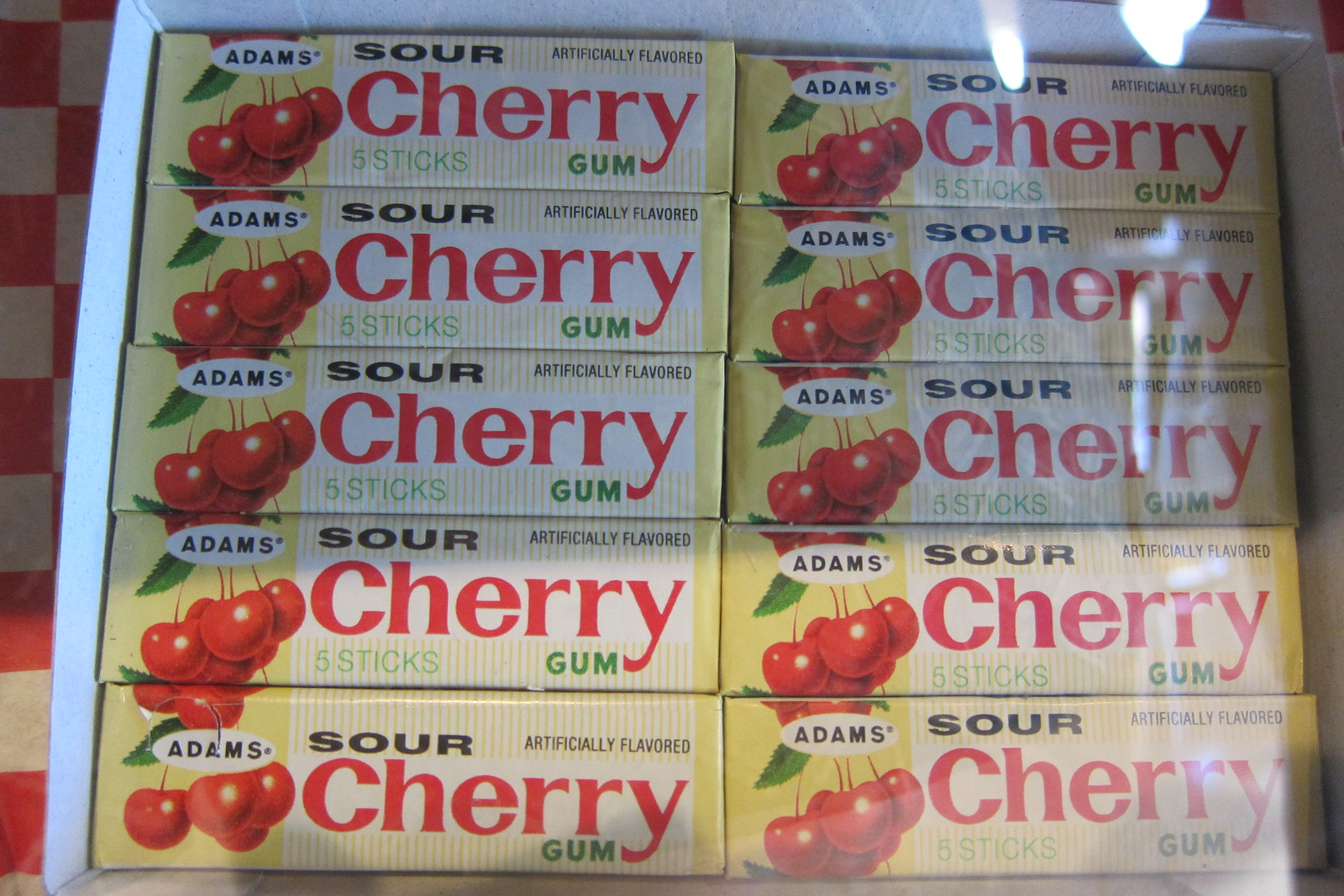The photograph captures a multi-pack of Adams Sour Cherry Gum, meticulously arranged within a white-edged carton, viewed from above through a clear plastic covering. Ten packs of gum are organized into two columns of five rows each. Each pack features a yellow box adorned with vivid black, red, and green lettering. Dominating the design, the word “SOUR” appears in bold, all-caps black font, followed by “CHERRY” in striking red capital letters, and beneath it, “GUM” in a prominent green font. Below the “CH” in “CHERRY,” it states “FIVE STICKS” in a less substantial font. The top right corner of the package indicates “ARTIFICIALLY FLAVORED.” The brand name "ADAMS" is displayed in black text within a white horizontal oval, which is superimposed on a vibrant cluster of red cherries with green leaves. The left side of the photograph displays a red and white checkered surface, and a noticeable glare on the right side implies the product is behind glass. The image epitomizes photographic realism, capturing the intricate details and vibrant colors of the product.